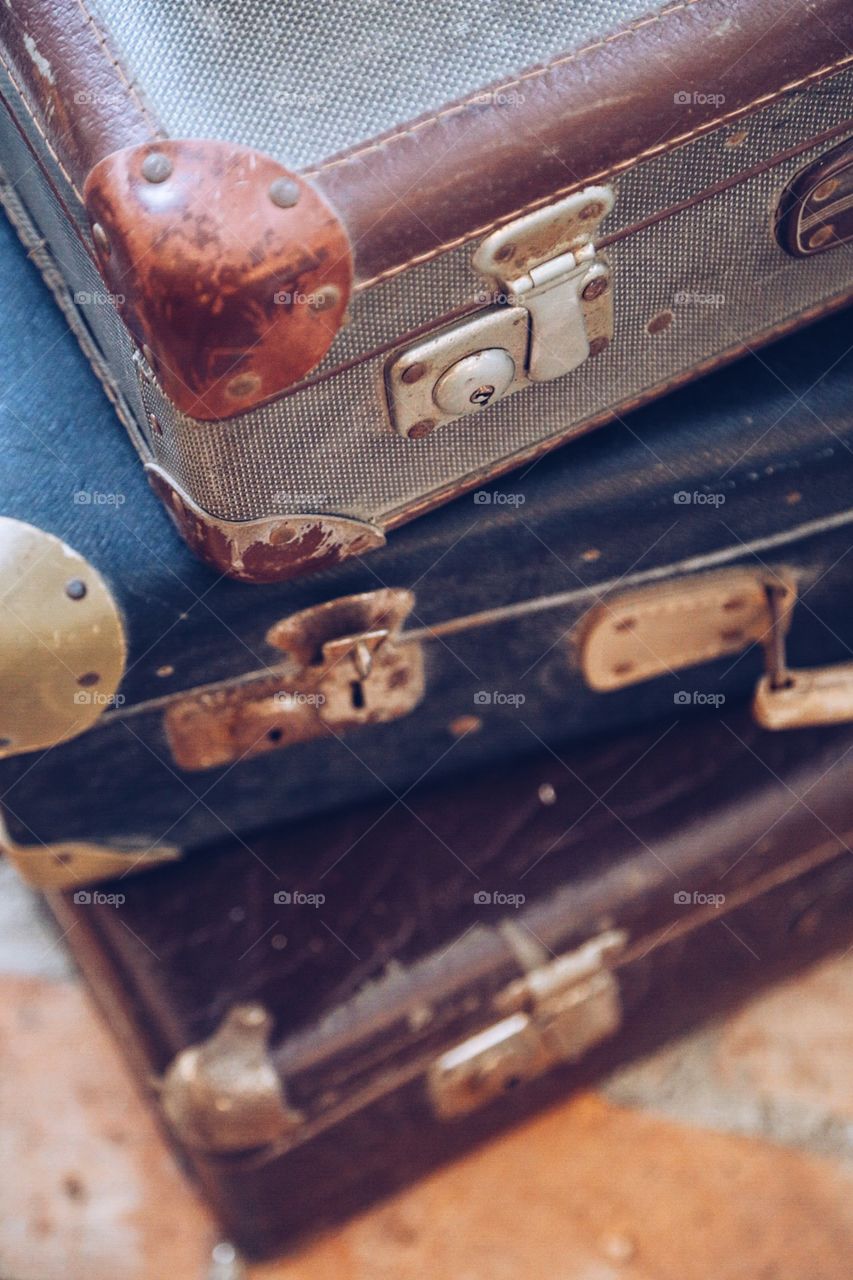The image depicts a stack of three weathered and old briefcases, positioned slightly off-center but mostly towards the top. The background appears to be a rough, possibly ground-like surface, suggesting the scene might be set in a garage or basement. Each briefcase shows significant signs of age, with rusty metallic parts and faded leather in shades of brown, gray, and blue. The bottom briefcase is dark brown with silver latches, resting on a tan, chipped table. The middle one is navy blue with gold latches, while the top one is gray with a dotted pattern, brown leather corners, and silver latches. A faint watermark with the text "F-O-A-P" and small camera icons in a diamond pattern is present across the image. The overall scene conveys a sense of nostalgia and the impression that these briefcases have been through numerous travels and adventures.